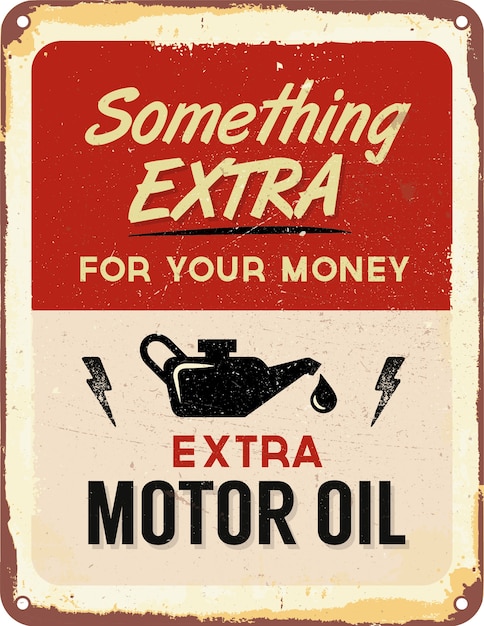This image is a vintage advertisement sign, likely for a mechanic shop, showcasing motor oil. The sign features a cream-colored, slightly faded background with a reddish-brown border that shows signs of wear and rust, particularly around the edges. Each of the four corners has a hole, presumably for mounting with screws.

At the top of the sign, there is a large, dull red rectangular box with rounded edges. Within this box, the text "Something EXTRA" is displayed. The word "Something" is in cream letters with only the 'S' capitalized, and "EXTRA" is in all capital letters, also in cream, and underlined in black.

Below this, on the cream background, there is an image of an oil can with a black lid and handle, depicted as if dripping an oil drop. Flanking the oil can are black lightning bolt symbols. Directly beneath the oil can, the text "EXTRA" is shown in red capital letters. Under this, in larger black capital letters, the words "MOTOR OIL" are prominently displayed.

The overall appearance is evocative of a classic advertisement designed for durability and visibility, possibly created and printed digitally, rather than hand-drawn. The detailed design elements and the worn look suggest its use in a historical or retro setting.